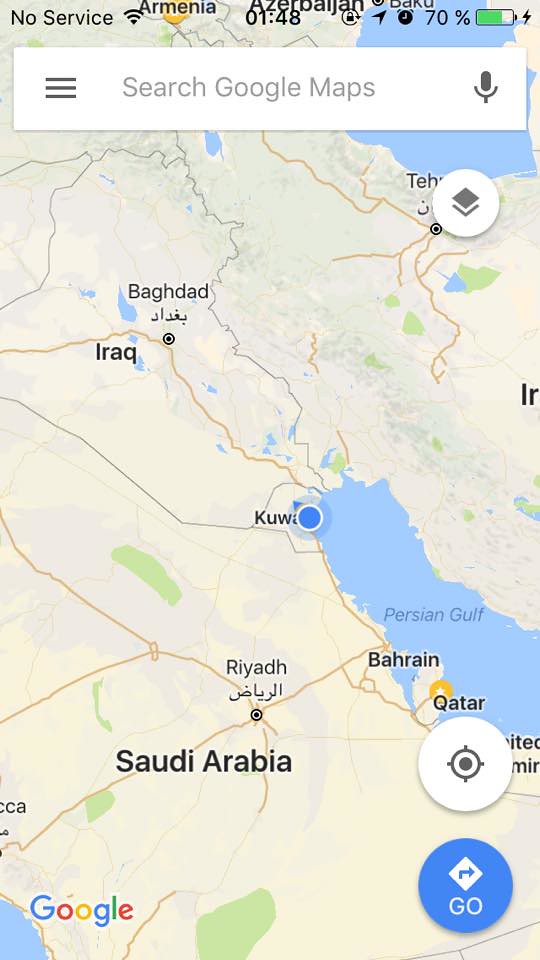The image depicts a Google Maps search screen on a mobile phone, showing a detailed map of the Middle East. At the top of the screen is a search bar with the gray text "search Google Maps," flanked by a three-bar menu icon on the left and a microphone icon on the right. Above the search bar, the phone's status is displayed, indicating "No Service," the time as 1:48, and the battery life at 70% in green. The map prominently features Kuwait marked with a blue pin. Surrounding regions are visibly labeled, including Iraq to the northwest with Baghdad, Saudi Arabia to the southwest with Riyadh, Qatar to the southeast, and the Persian Gulf to the east. Additional locations such as Tehran, Armenia, and Azerbaijan are also labeled. At the bottom left is the Google logo, and the bottom right corner features a blue circle labeled "Go," with a diamond containing a blue arrow.